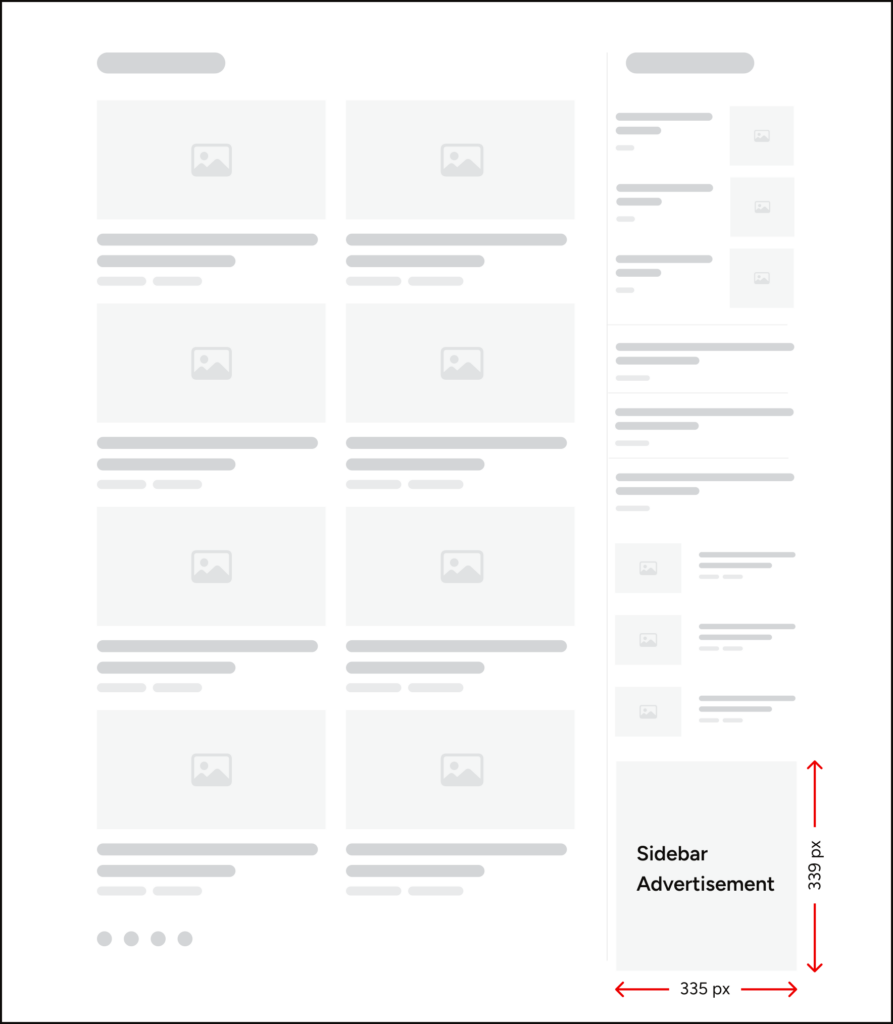This image depicts a skeletal design of a website template, notably lacking informational content. At the bottom right corner, two prominent labels, "Sidebar" and "Advertisements," are prominently displayed in dark black text. Adjacent to these labels, the bottom edge features a numerical designation "335 PX," with red arrows flanking it, extending both left and right, indicating adjustable width. Similarly, on the right side, a fittingly rotated indicator reads "339 PX," with the same red arrows suggesting adjustable height.

Moving upwards, several smaller boxes adorned with photo icons are visible, each accompanied by a set of horizontal lines extending to the right. The top two lines are in a darker gray, while the third one beneath them appears in a lighter gray hue. Dominating the top center, a sequence of eight small square boxes is arranged in a grid-like pattern, consisting of two columns with two boxes each, repeating across the section.

Further enhancing the geometric layout, thick oval-shaped rectangular elements occupy the top left and top right corners, lending a bold, rounded aesthetic to the boxy design elements. The overall impression is a clean, minimalistic website framework emphasizing content blocks and adjustable sections.